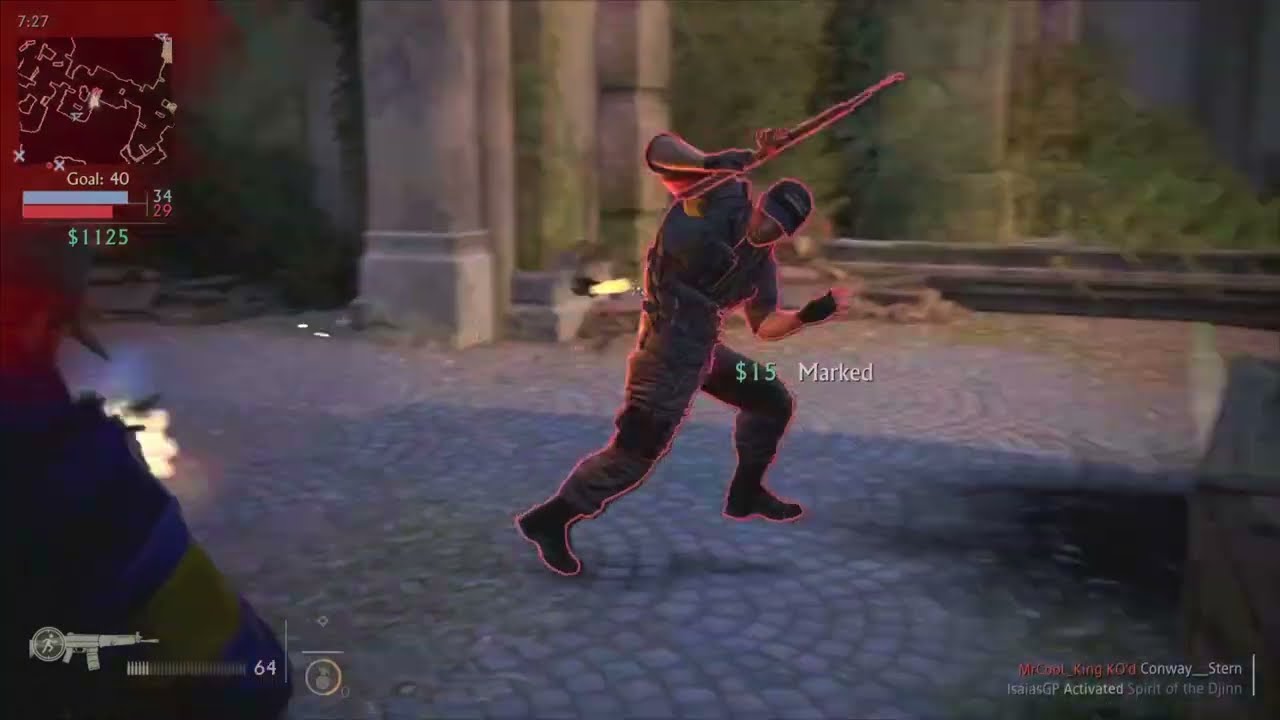The image depicts a game interface with various elements. Dominating the center is a man clad in green army fatigues and a cap, positioned as if he's evading something. He stands on a ground made of tiny, gray cobblestones, amidst columns and a stone wall that has some green plants. The man has his right hand raised, holding a long pistol at an angle above his head, while he slightly bends his body to the right. His left leg is bent forward, giving the impression of movement, as if he's either running or crouching. His left hand is in front, bent at the elbow, adding to the sense of alertness. 

At the top left corner of the screen, the game displays the text "Goal 40 $1,125." Additionally, "$34" in blue and "$29" in red are noted, possibly indicating scores or objectives. A timer or game progress counter marked "727" is also visible. In the bottom left, there's an icon of a machine gun accompanied by the text "$64," likely relating to ammunition or resources. The right bottom corner features text referencing "King Conway Stern Activated Spirit of the Djinn," hinting at either a character name or a game chapter. The overall scene suggests the man is prepared for combat within a detailed, immersive environment.